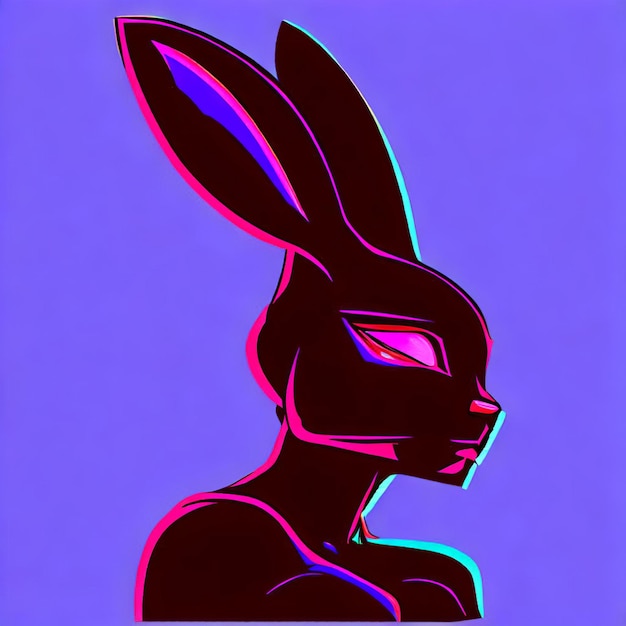This graphic digital art image features a striking silhouette set against a neon purple background. The central figure is a unique amalgamation of a human female form and a bunny, predominantly shown from the bust up. The humanoid bunny is oriented to the right, with unmistakably long, black ears; the left ear is edged in vibrant neon green, while the right ear is accented with neon pink. Neon pink also outlines the rabbit's profile, defining the facial features such as the eyes and nose with luminescent clarity. A pink line traces the neck and arms, extending downwards to suggest the contours of a woman's upper body. The overall design is minimalist yet modern, characterized by sharp, clean divisions of color that emphasize the surreal fusion of human and rabbit elements. The interior of the silhouette is a deeper purple, providing a stark contrast to the bright, neon highlights, making this artwork a bold and captivating visual experience.